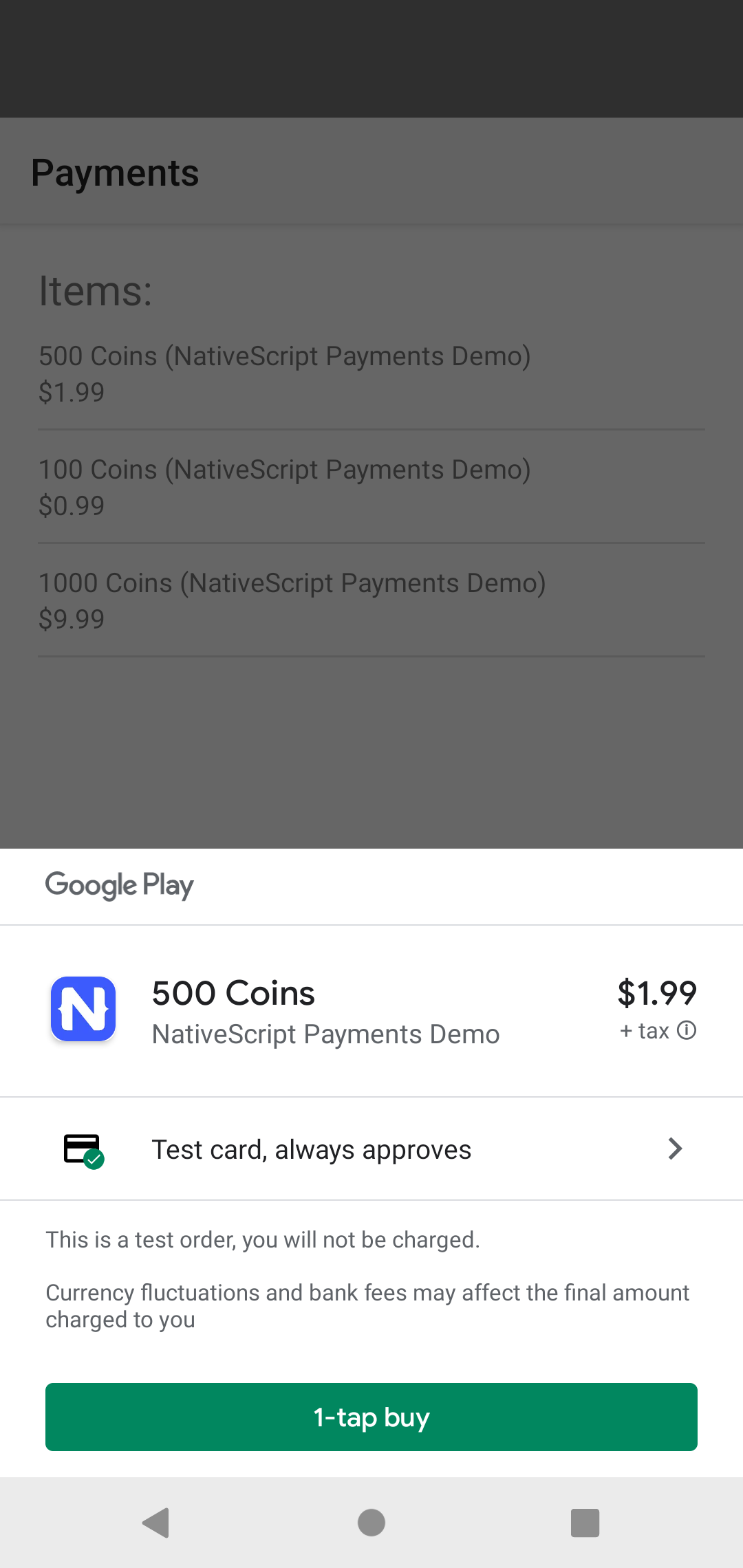The image displays a payment interface pop-up with several elements detailed below:

- **Top Section**: 
  - The upper portion of the interface has a shaded gray overlay due to a pop-up obscuring it. The topmost part features a darker gray border.
  - Despite the shading, it appears to have a white background. 
  - The word "Payments" is prominently displayed in black.

- **Item List**:
  - Beneath a thin gray separator line, the list of items begins.
  - The first item listed is "500 coins," written in gray.
  - In parentheses, it specifies: "Native Script Payments Demo, $1.99."
  - This description is followed by another thin horizontal gray line.
  - The second item listed is "100 coins," also described in parentheses as: "Native Script Payments Demo, $0.99."
  
- **Pop-Up Details**:
  - The pop-up itself is white, matching the background color. 
  - In the upper-left corner of the pop-up, "Google Play" is written in gray. 
  - Another thin horizontal line runs beneath this text.
  - A blue square icon with a white capital "N" is present, symbolizing Native Script.
  - Adjacent to the icon is the text "500 coins," written in bold black.
  - Directly below this, it reiterates: "Native Script Payments Demo."
  - To the side, the price "$1.99" is displayed with a plus sign and the word "tax." Next to this, a gray circle contains a gray "i" indicating information.

- **Payment Method**:
  - Below another thin horizontal line, the text "Test card, always approve" appears in black with a right-pointing arrow.
  
- **Additional Information**:
  - Another horizontal line separates the following notice, in black: "This is a test order. You will not be charged. Currency fluctuations and vague fees may affect the final amount charged to you."
  - The phrase "Native Script Payments Demo, $1.99. Currency fluctuations and vague fees may affect the final amount charged to you." is repeated.

- **Action Buttons**:
  - The bottom of the interface features a green rectangle and a white rectangle.
  - The white rectangle contains the text "1-TAP BUY."

This detailed description outlines the layout and content of the payment interface depicted in the image.